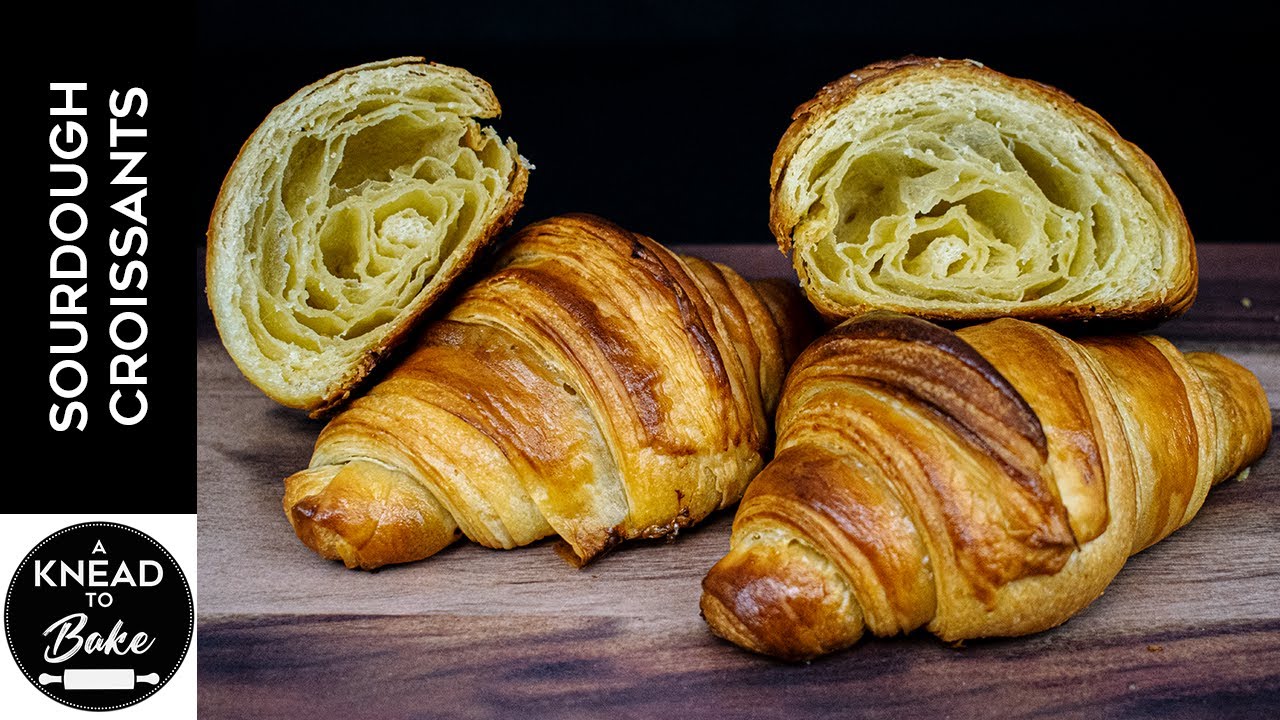This close-up promotional image showcases four well-baked sourdough croissants arranged on a dark wooden surface against a completely black background. The two whole croissants are glistening with a rich, golden-brown hue, while the two halves are meticulously placed atop the whole ones, exposing their airy, flaky interiors filled with delicate swirls and pockets. On the left side of the image, running vertically, the text "Sourdough Croissants" is prominently displayed in white. Beneath this, there is a black circle with a white beaded border containing the phrase "Knead to Bake" in white text, accompanied by a rolling pin icon. This elegant layout and detailed presentation emphasize the quality and appeal of the croissants, making them perfect for an advertisement.